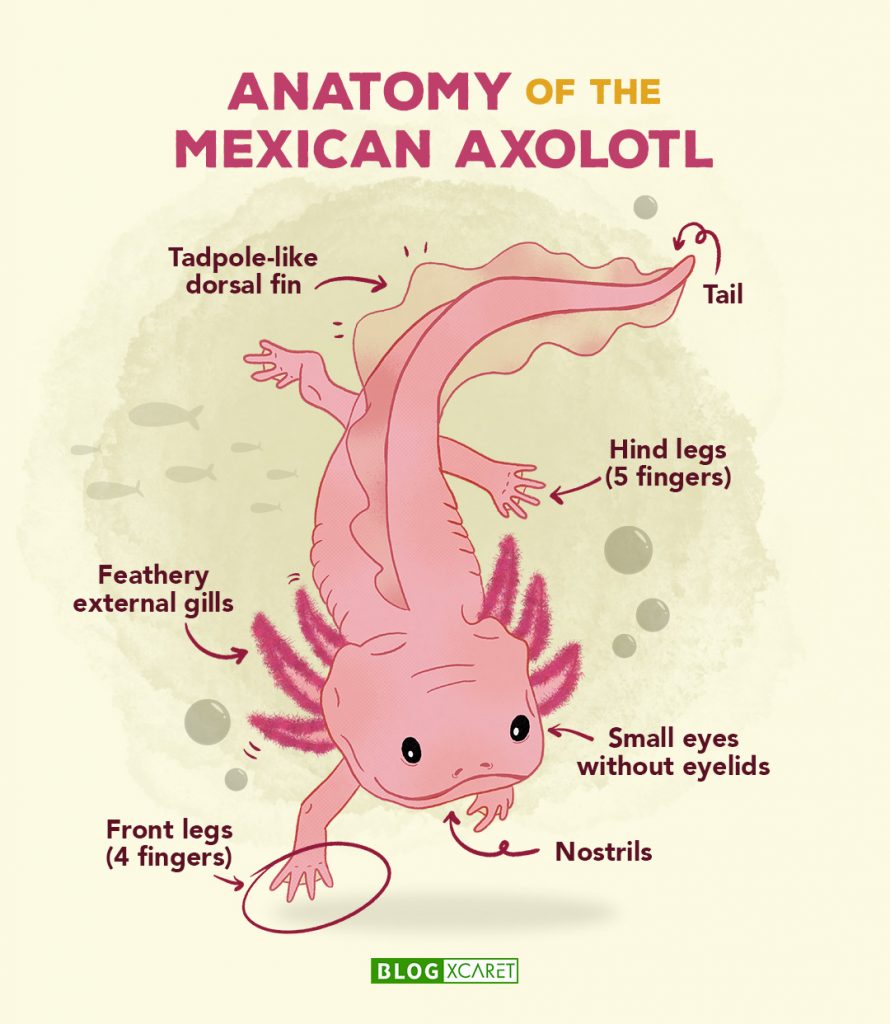The illustration, titled "Anatomy of the Mexican Axolotl" in pinkish-red lettering, is a detailed and instructional depiction of the Mexican axolotl, a type of salamander. The axolotl itself is rendered in pink, with its body positioned vertically in the center of the image. Its face looks slightly down and to the right, while its tail curls upward to the top right. The background behind the axolotl is a watery greenish hue with bubbles and fissures, contrasting a beige overall poster background.

Various anatomical features of the axolotl are meticulously labeled with arrows and text. The small eyes are marked with "small eyes without eyelids," while the nostrils are simply labeled "nostrils." Its feathery, dark pink external gills extend from both sides of its head. The axolotl has four front legs with four fingers each, and its hind legs, which are labeled "hind legs, five fingers," have five fingers each. The dorsal fin on its tail, described as "tadpole-like," is another key characteristic pointed out in the illustration.

At the bottom of the poster, green text in relief reads "blog Xcaret," with the word 'blog' embossed and the letters of 'Xcaret' reversed in color scheme relative to the cream and green colors used. The overall visual setup effectively communicates the unique anatomy of this fascinating creature.